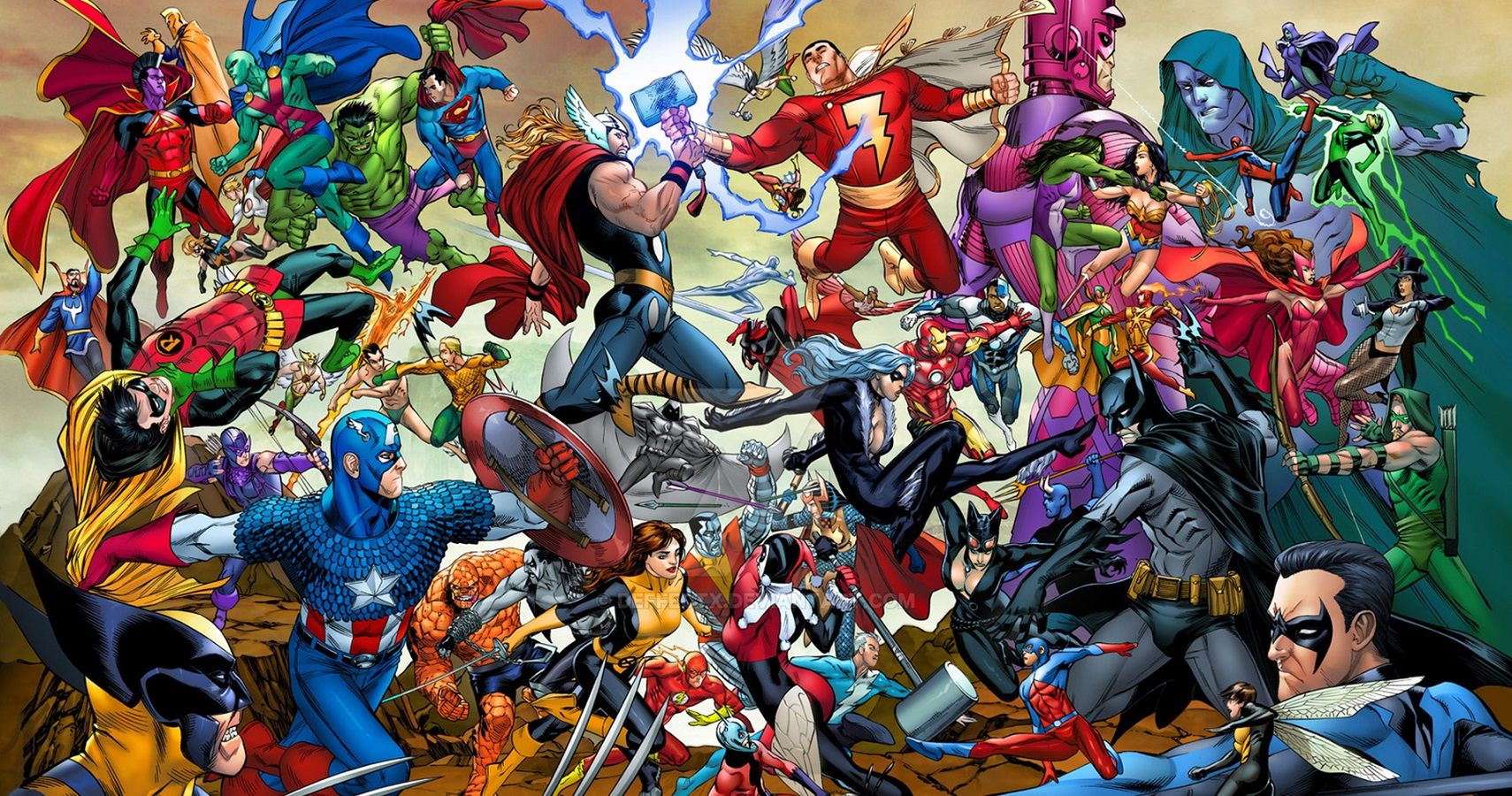This vibrant comic book-style illustration depicts an intense battle between a diverse group of superheroes from both Marvel and DC universes. In the bottom left corner, Wolverine, with his iconic claws, stands next to Captain America, who is prominently wielding his red, white, and blue shield. Above them, Batman is seen strategically positioned. Toward the middle of the scene, Thor, brandishing his mighty hammer Mjölnir with lightning emanating from it, is engaged in a fierce fight with the Flash, recognizable by his red suit and lightning bolt emblem. Dominating the top of the image, the Hulk, depicted in green and purple, shows his immense strength by lifting Superman high above the chaotic fray. Flying through the air above them is Robin, adding to the dynamic and frenetic energy. Scattered throughout the scene are other heroes, including Wonder Woman and Green Lantern, all locked in combat. The detailed illustration captures a climactic showdown with vibrant, colorful depictions of these iconic characters, each illustrating their unique powers and characteristics.